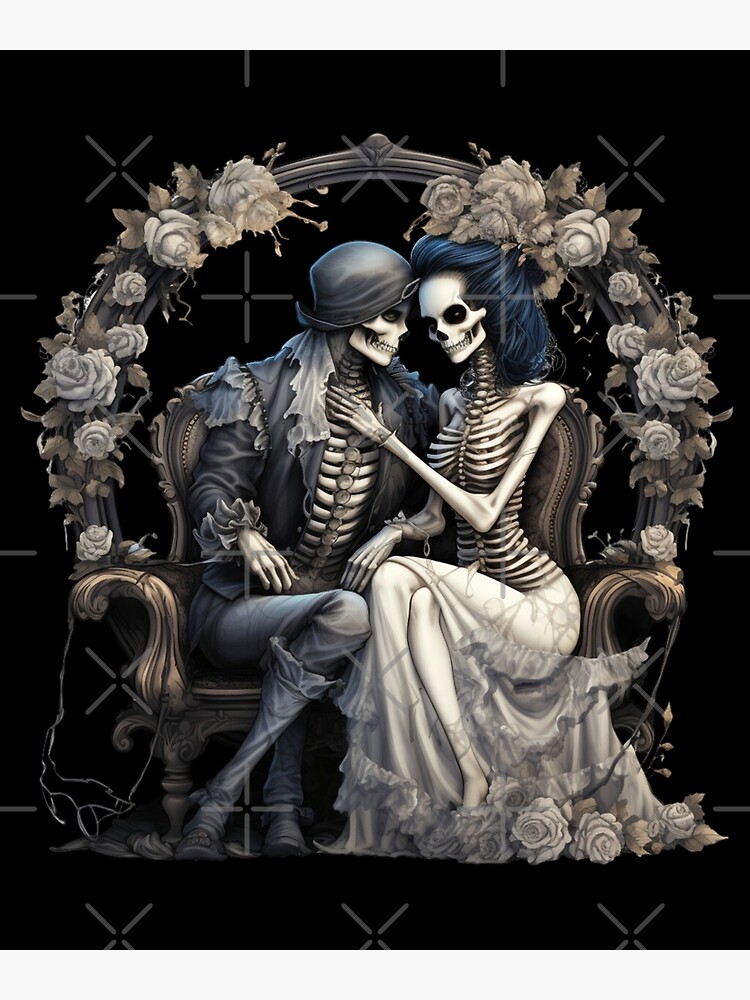This image depicts an intricately detailed scene of two skeletons seated on a brown sofa, set against a stark black background adorned with watermark X's and pluses. The skeleton on the right, representing a female character, has long, dark blue hair artistically tied up, adorned with flowers and gothic touches. She wears the bottom half of a white wedding gown, the fabric elegantly cascading from her waist. Her skeletal form is starkly depicted, with her left arm tenderly draped across the male skeleton’s chest, pulling them close together as if preparing for a kiss. On the left, the male skeleton presents a rugged, biker aesthetic, dressed in a black leather jacket, jeans, and boots, with his skull partially covered by a leather cap. His ribcage and chest are fully exposed, matching the raw skeletal display of the female. Both figures are framed by a wreath of white roses that arches gracefully from one arm of the sofa to the other, encapsulating the romantic, yet eerie essence of the scene, reminiscent of a gothic, post-apocalyptic nuptial portrait.